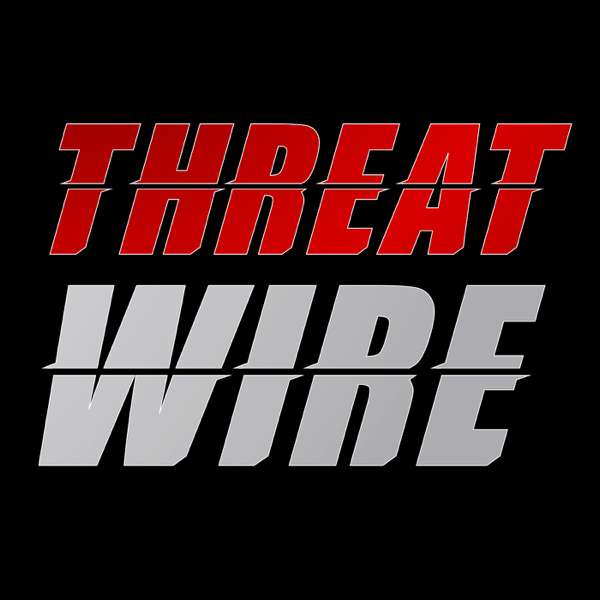The image is a simple yet striking design featuring a square black background. Positioned at the top center is the word "THREAT" in bold, capitalized, red letters, slightly italicized to the right. A black horizontal line bisects each letter, separating them into two pieces. Directly beneath "THREAT" is the word "WIRE," written in bold, capitalized, very light gray letters, also slightly italicized to the right and bisected by a horizontal black line. The black lines create a visual disruption, giving the letters a split or fragmented appearance. There is no additional text or imagery in the image.